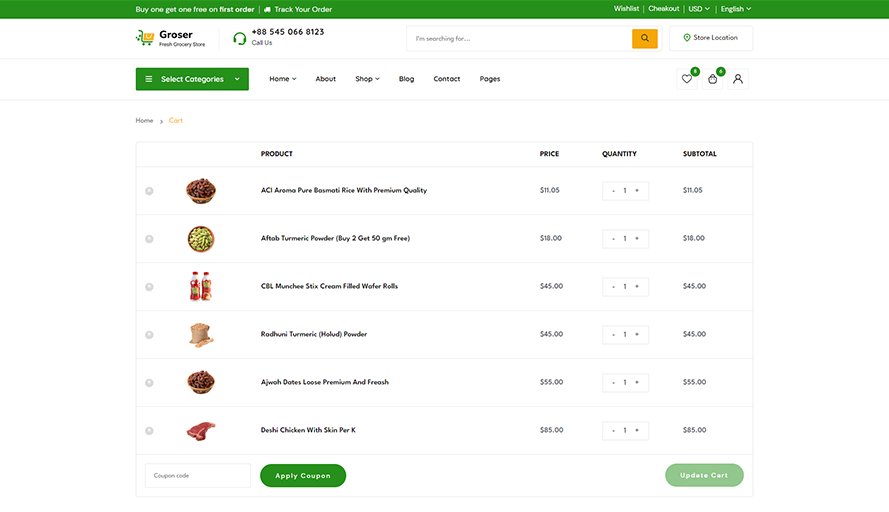The image depicts a detailed screen of a grocery store's online ordering website, specifically the cart section featuring items chosen by the user. The screen is structured with prominent details to assist shopping processes:

**Top Banner**: A green banner at the top displays a promotional message in white text, offering a "Buy One Get One Free" deal on the user's first order. To the right of the banner are multiple interactive options including:
- **Track Your Order**: A feature to monitor order status.
- **Wish List**: An option for users to add desired products for later purchase.
- **Checkout Button**: Directs the user to finalize their purchase.
- **Currency Selector**: Currently set to USD, allowing users to change the preferred currency.
- **Language Selector**: Currently set to English, enabling language change for the interface.

**Secondary Row**: Below the banner is a secondary strip containing:
- **Customer Service Phone Number**: Accompanied by a phone icon, the text "Call Us" directs users to contact customer service via phone.
- **Search Box**: Users can enter product details to search the store’s inventory.
- **Store Location Button**: Helps users find physical store locations.

**Category Selection**: A drop-down menu is available to filter products by categories.

**Cart and Favorites Icons**: To the right, two additional icons indicate the number of items in the shopping cart and favorites (heart icon), along with an account information icon.

**Main Cart Section**: The middle part of the screen lists six selected items, each accompanied by:
- **Product Image**: Visual representations of the items.
- **Description**: Brief details about each product.
- **Price**: The cost per unit.
- **Unit Price**: Breakdown of cost per unit quantity.
- **Quantity**: Number of units ordered.
- **Subtotal**: Total cost for each item based on quantity.

**Bottom Section**: At the bottom left corner, there is a:
- **Coupon Code Box**: Textbox to enter promotional codes.
- **Apply Button**: To apply the entered coupon to the order.

This comprehensive setup provides users a seamless and efficient online grocery shopping experience.